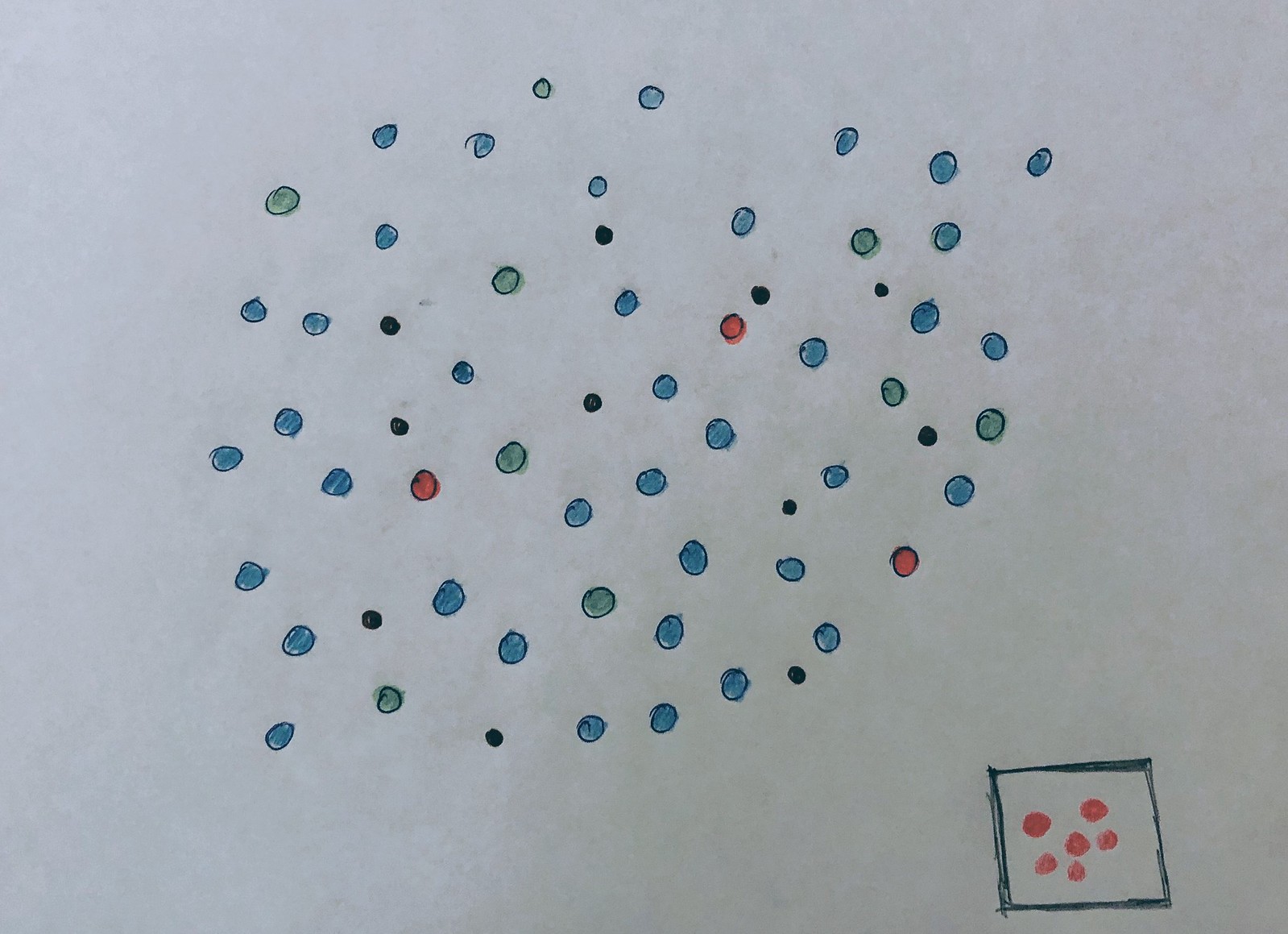The image showcases an array of small, irregularly-shaped dots against a gray background. These dots, varying in form, are plentiful and scattered across the entire scene. They appear in a range of colors, including red, green, blue, and a few dark hues. Arranged in what seems like a continuous line rather than a spiral, the dots are unevenly spaced. The background, resembling a sheet of paper, is oriented horizontally. In the bottom right corner of the paper, a small square drawn with grayish ink contains six pink stones or pebbles. These stones are distinctly decorative and visually appealing, contributing an element of contrast to the overall composition.